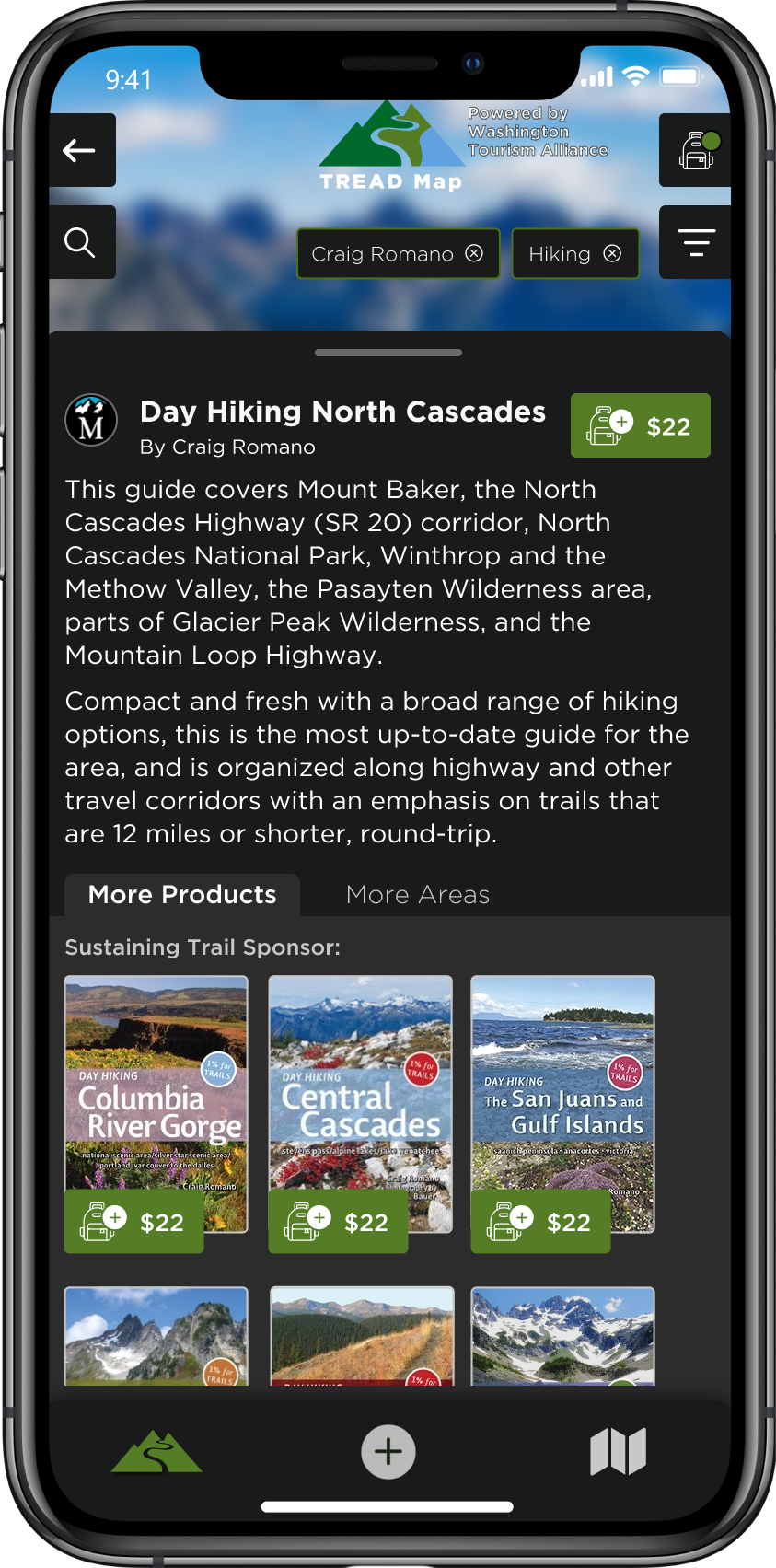The image showcases a vertically rectangular frame featuring a cell phone displaying an app. The app interface presents a detailed hiking guide titled "Day Hiking North Cascades" by Craig Romano, accompanied by a prominent green price button indicating "$22." The guide boasts coverage of various regions including Mt. Baker, the North Cascades Highway, the State Road 20 Corridor, North Cascades National Park, Winthrop, the Methow Valley, the Pasayten Wilderness Area, parts of the Glacier Peak Wilderness, and the Mountain Loop Highway. This compact and up-to-date guide is praised for offering a wide range of hiking options, particularly focusing on trails that are 12 miles or shorter in round trip length. The guide is organized by highways and travel corridors to facilitate easy navigation. At the bottom of the app interface, users can toggle between two tabs: the currently active "More Products" tab and the "More Areas" tab. Under the "More Products" tab, the section features images of various trail sponsors, complete with locations and pricing details.